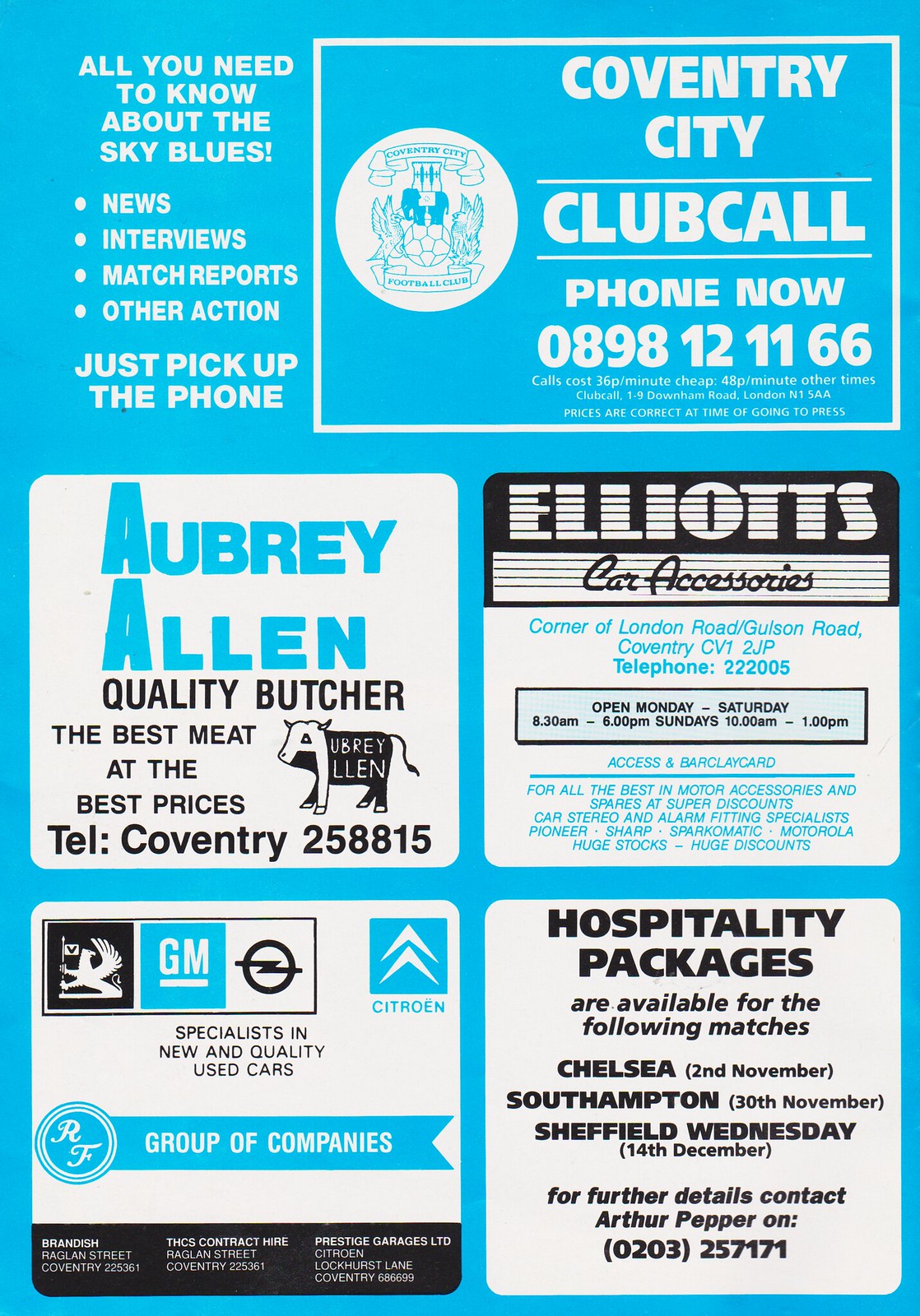This flyer, set against a blue background, provides comprehensive information about Coventry City Club Call. It highlights that you can get news, interviews, match reports, and other action regarding “The Sky Blues” by calling 0898-1211-66. The call costs are 36 pence per minute during cheap times and 48 pence per minute at other times. Located at 1 Downham Road, London, N15AA, the flyer boasts accurate pricing at the time of printing. 

In addition to the main advertisement, the flyer features four white-panel ads. These include Aubrey Allen Quality Butcher, known for the best meats at the best prices, contactable via Coventry 258-8815; Elliott’s Car Accessories located at the corner of London Road and Gulsun Road in Coventry, with a contact number of 222-005; GM Specialists in New and Quality Used Cars, displaying multiple car logos including Citroen within the RF Group of Car Companies; and details regarding hospitality packages available for matches against Chelsea on November 2nd, Southampton on November 30th, and Sheffield Wednesday on December 14th. For more information, contact Arthur Pepper at 020-3257-171.